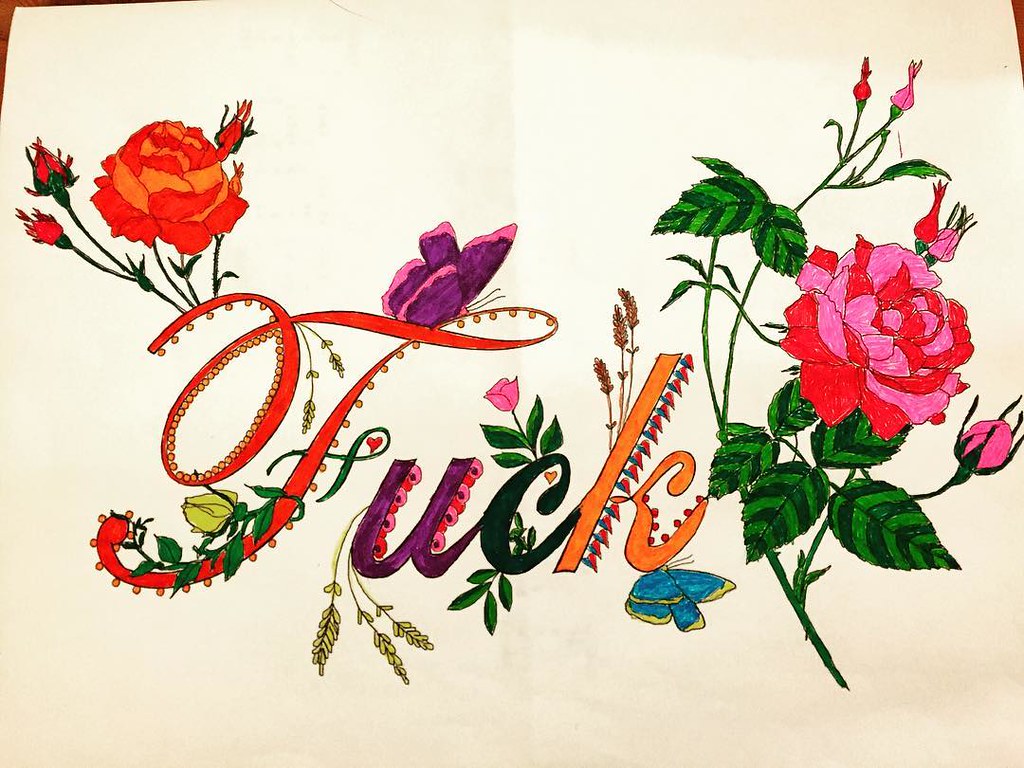The image is an ornate piece of artwork displayed on white or possibly off-white paper. It prominently features the word "F-U-C-K" in vibrant, handwritten script, with each letter rendered in a different color: the F is red, the U is purple, the C is green, and the K is orange. Surrounding and intertwining through the letters are a variety of flowers and stems, contributing to a decorated and intricate design. The flowers vary in color, including orange, red, and pink blossoms with green leaves and stems. Also integrated into the artwork are several butterflies, with a notable giant butterfly perched atop the F, and another blue and green butterfly near the bottom of the K. There are some green vines and buds adding to the lush, garden-like aesthetic. Additionally, a small heart is situated by the F, enhancing the detailed and elaborate look of the composition. The entire piece appears to be meticulously created with colored pencils or markers.